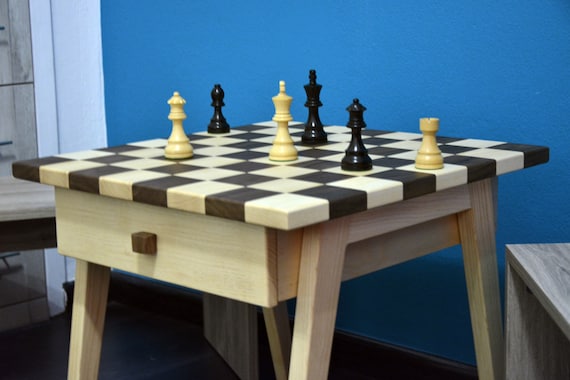The image features a square table with a light-colored wood base, including a drawer with a square handle, and diagonally angled legs connected by a bar beneath the tabletop. The tabletop itself is designed as a black-and-white checkered chessboard. Placed on this table are six chess pieces: three white and three black, including a king, queen, and various other pieces. The scene is set indoors against a bold royal blue wall. To the side of the table is a smaller piece of gray furniture. Further details include a gray-brown file cabinet with silver handles and a white section of trim in the background, contributing to the overall setting which resembles a cozy nook designed for chess games.